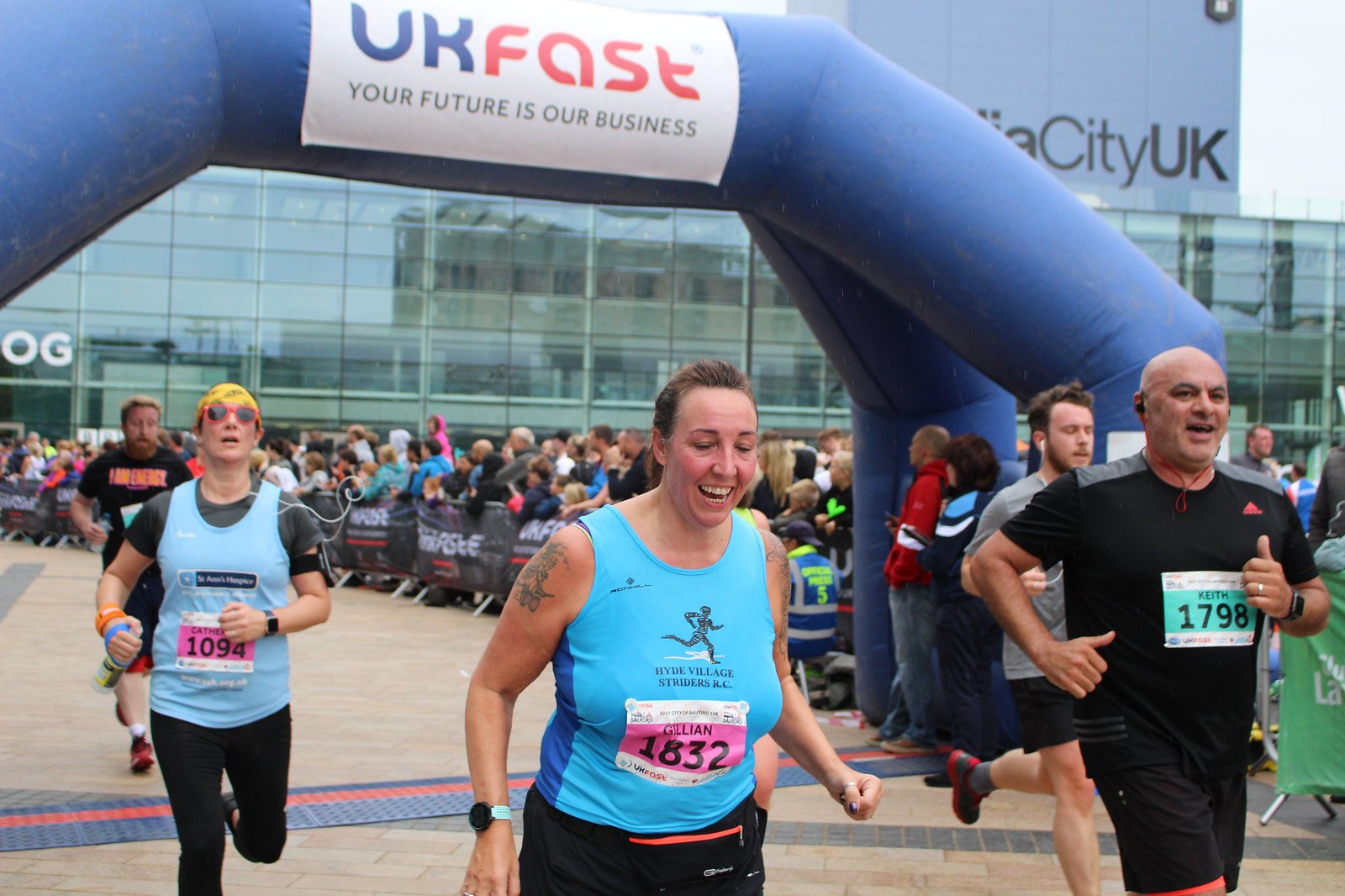This photograph captures the vibrant scene of a marathon where participants are running past the finish line, an eye-catching blue inflatable arch that reads "UK FAST" in blue and red, and "Your future is our business" in black. Among the runners, there's a noticeable middle-aged woman with brown hair, wearing a blue top that reads "Hyde Village Striders RC" and a name card labeled "Gillian 1832." She is flanked by other marathoners, including two men and one other woman who have already crossed the finish line, and a man in a black shirt with blondish hair and a brown beard about to cross. The background features a striking mirrored glass building, reflecting a yellow structure across the street, and above it, a partially obscured sign that reads "City, UK.” Spectators line the sides of the road behind barricades adorned with sponsors' signs and flags, cheering the runners on.